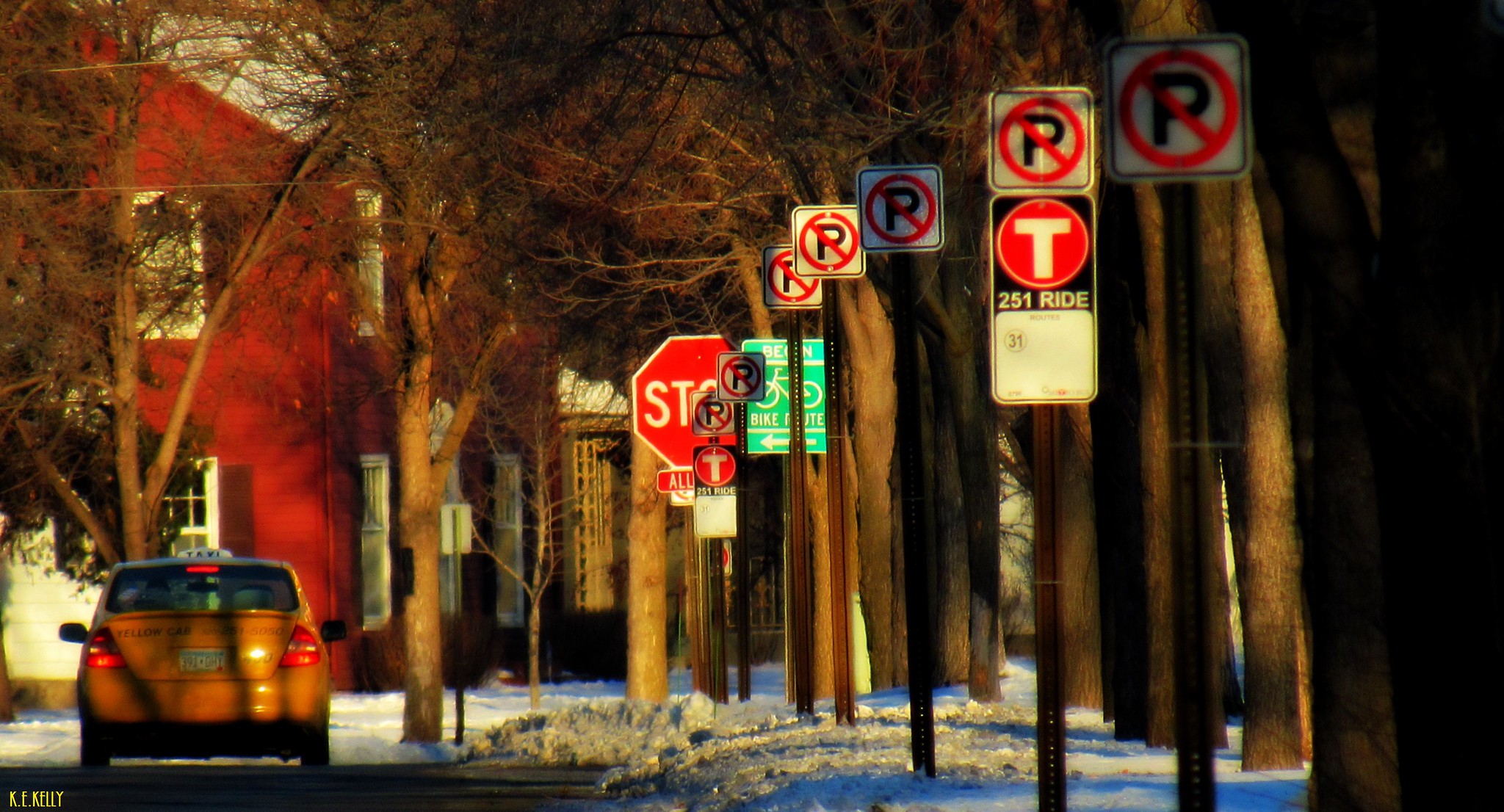This photograph, taken on a sunny winter day downtown, captures a busy street scene. The main focus is on a series of about seven white "No Parking" signs with bold black "P"s crossed by red circles, aligning the snow-covered ground. Interspersed among these is a bigger sign with a white "T" in a red circle, a black background, and "251 Ride" in white font at the bottom. The right side of the image features thick brown tree trunks, bare from the winter cold. In the foreground on the far left, a dark burnt-yellow taxi cab is driving away down the black road, showcasing "TAXI" written in black on a white panel. In the background, there is a two-story red brick building with black shutters and white-framed windows, partially obscured by the line of trees and signs. The taxi’s rear displays yellow lettering, possibly reading "K-L" or "Kelly." The overall scene is a vivid depiction of a typical downtown winter day, accentuated by the clear blue sky, snow-blanketed ground, and leafless trees.